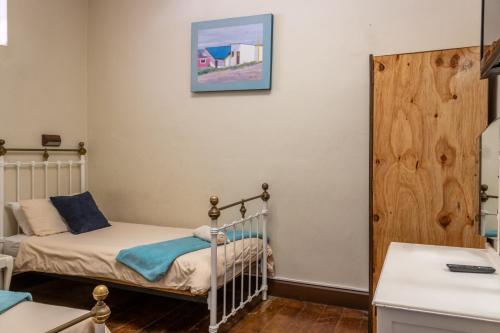The photograph showcases a simple, old-fashioned bedroom that could be a child's room, a dormitory, or a hostel room. The room features two twin beds with white metal frames accented with brass fixtures. Each bed is made with off-white linen sheets, complemented by white and off-white pillows, and a turquoise blue throw blanket at the foot. A navy blue accent pillow adds a pop of color. The room has wood flooring and an overall plain, off-white interior. On the back wall, there is a painting in a blue frame depicting a white building, which complements the room's blue accents. To the right of the frame, a white countertop or dresser with a mirror is visible, adjacent to a natural wood panel, possibly covering a door or part of a closet. A sliver of a window in the upper left allows a glimpse of natural light into the otherwise sparse room.